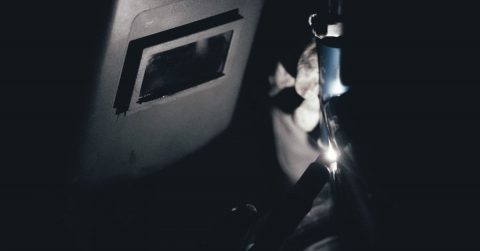In this close-up image, set against a completely black background, a welder is captured in the midst of their craft. Positioned on the left side of the frame, the subject is wearing an all-black welding mask equipped with a small, darkened viewing window, possibly made of glass or hard plastic. This protective screen shields their eyes from the intense light generated during welding. The welder appears to be kneeling, focusing intently on their task. Clad in protective gloves, they manipulate a tool in their right hand that emits a bright, white light—suggesting it could be a specialized torch or laser used in welding. Although the precise nature of the material being welded is obscured by the darkness, the intensity and concentration of the welder's posture indicate a meticulous and careful process.